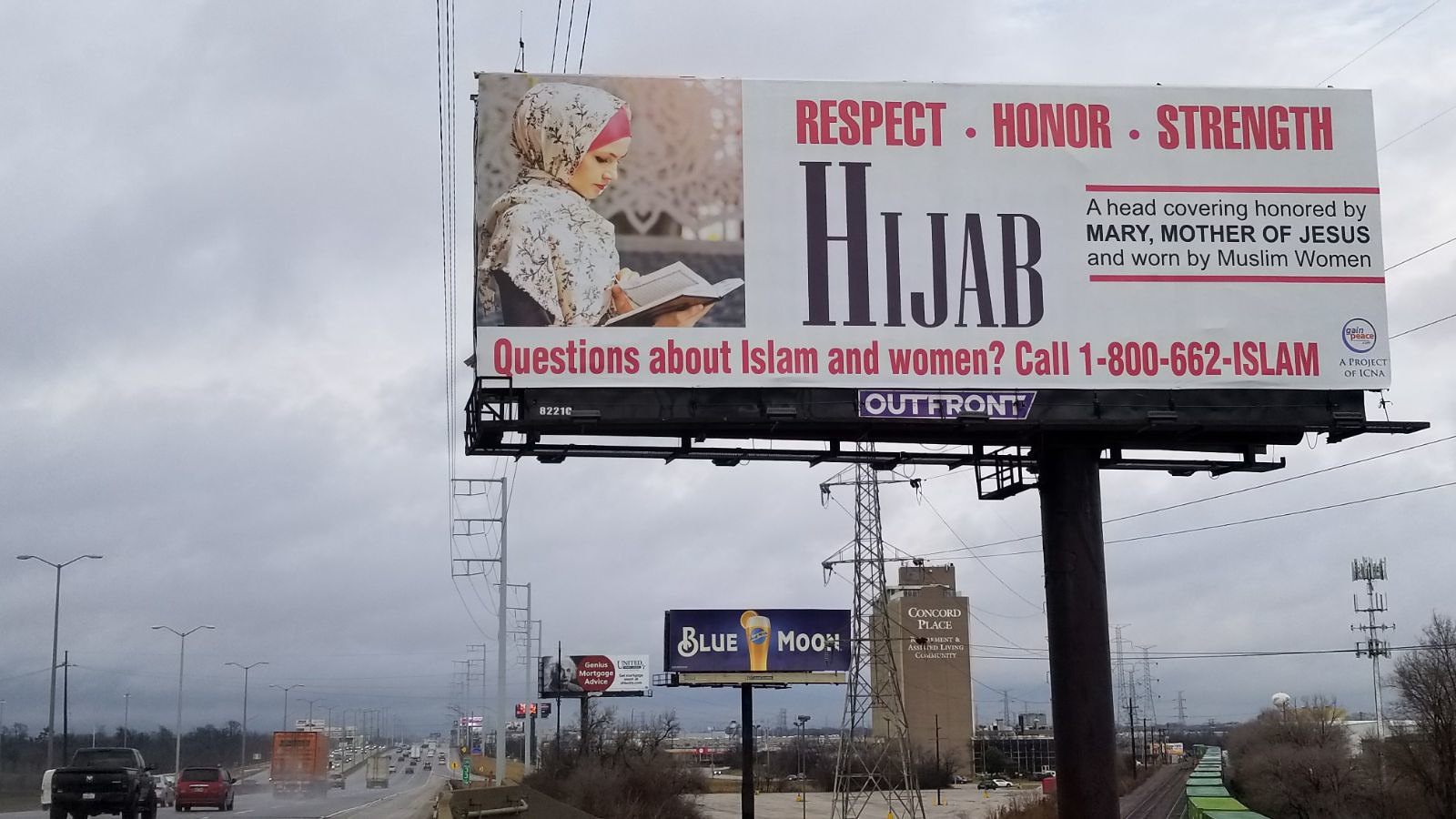In this outdoor photograph, three billboards dominate the scene against an overcast gray sky with some visible cloud formations. The main focus is a large billboard that features the text: "Respect, Honor, Strength, Hijab. A head covering honored by Mary, Mother of Jesus, and worn by Muslim women." The billboard includes a contact number for questions about Islam and women. The billboard's brand is "Out Front," and in its upper left corner, there is an image of a woman wearing a hijab, reading a book while seemingly seated. Beneath this main billboard is a smaller one advertising Blue Moon Beer. Adjacent to the billboard on the lower left corner of the photo is a large expressway. Several electrical posts and wires surround the scene, indicating an urban setting.